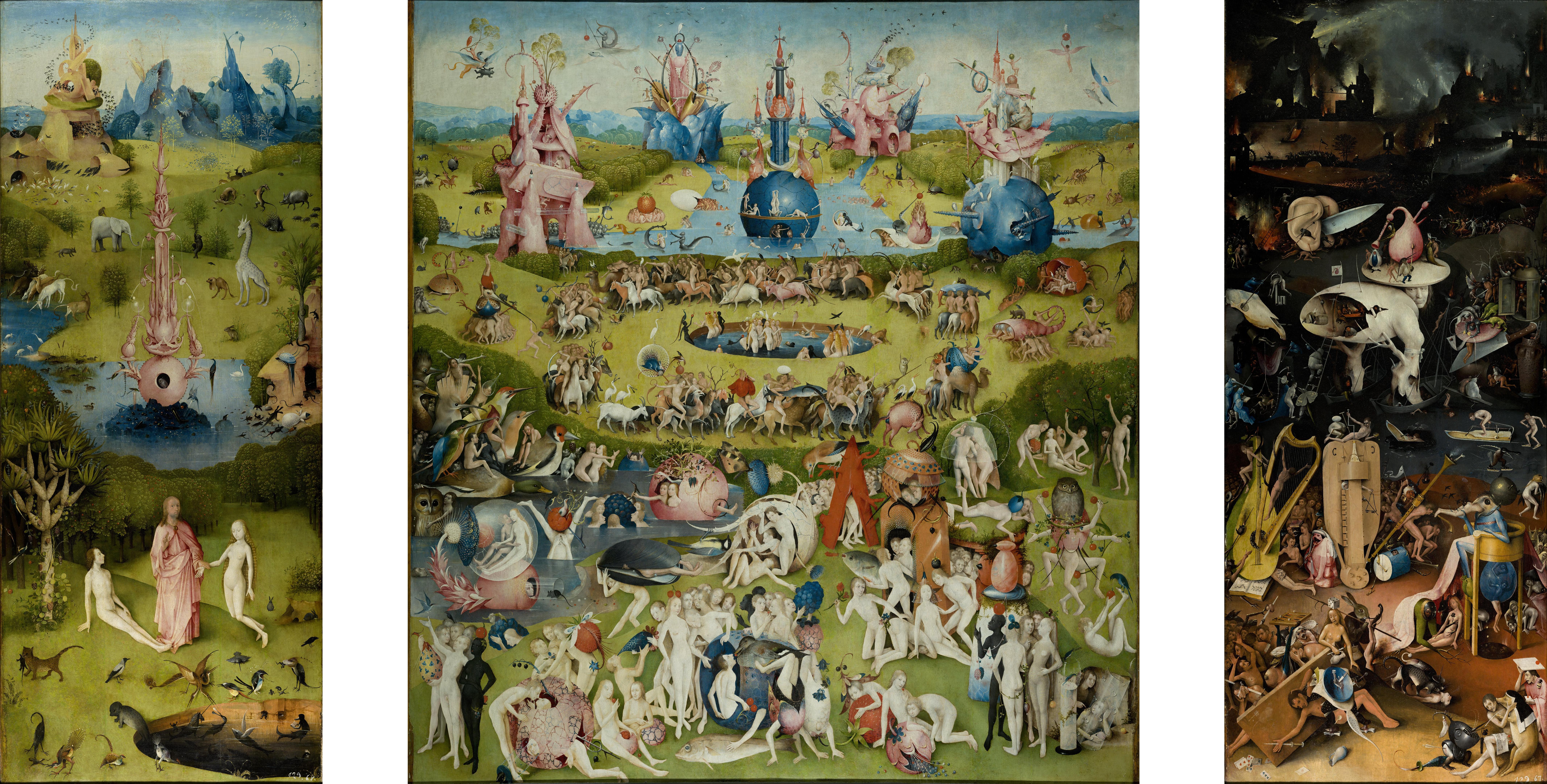This intricate triptych is a rectangular artwork consisting of three vertical panels with the central one being slightly larger. The composition showcases a rich tapestry of life, blending human figures, animals, and fantastical structures. The scenes are imbued with a kaleidoscope of colors, including vibrant greens, blues, pinks, browns, yellows, and blacks, creating a vivid and bustling narrative that unfolds from left to right.

Starting with the left panel, the scene is set in a bright, verdant landscape, where a few people and animals coexist amidst whimsical castles and curious objects. This section appears relatively serene and is drawn in light hues of green and blue, establishing a morning-like or early day ambiance.

The central panel, which is the most detailed and expansive, illustrates a densely populated and dynamic scenario. The bottom third is teeming with numerous naked figures, mingling and engaging with one another. Above them, animals form a circle around a central pond wherein more people are gathered. The midsection features otherworldly castles with spiky towers set within a small lake, casting an enchanting spell over the scene. The color palette here continues the vibrant theme, with interspersed shades of white and blue in the sky above, highlighting a sense of daylight and liveliness.

In stark contrast, the right panel transitions to a considerably darker theme, hinting at a nighttime or end-of-day scenario. The hues shift to include more browns and blacks, and the overall image seems almost mine-like, filled with random objects and scattered people. The sky in this section is dark, accentuating a somber and perhaps celestial atmosphere. Imagery of chaos is evident, with scenes suggesting conflict or aftermath, such as arrows and dying figures, and buildings that seem to be engulfed in flames.

Altogether, this artwork artfully captures the nexus of human experience and imagination, juxtaposing moments of calm and tranquility with scenes of turmoil and darkness, hinting at a narrative arc that spans from morning to night.